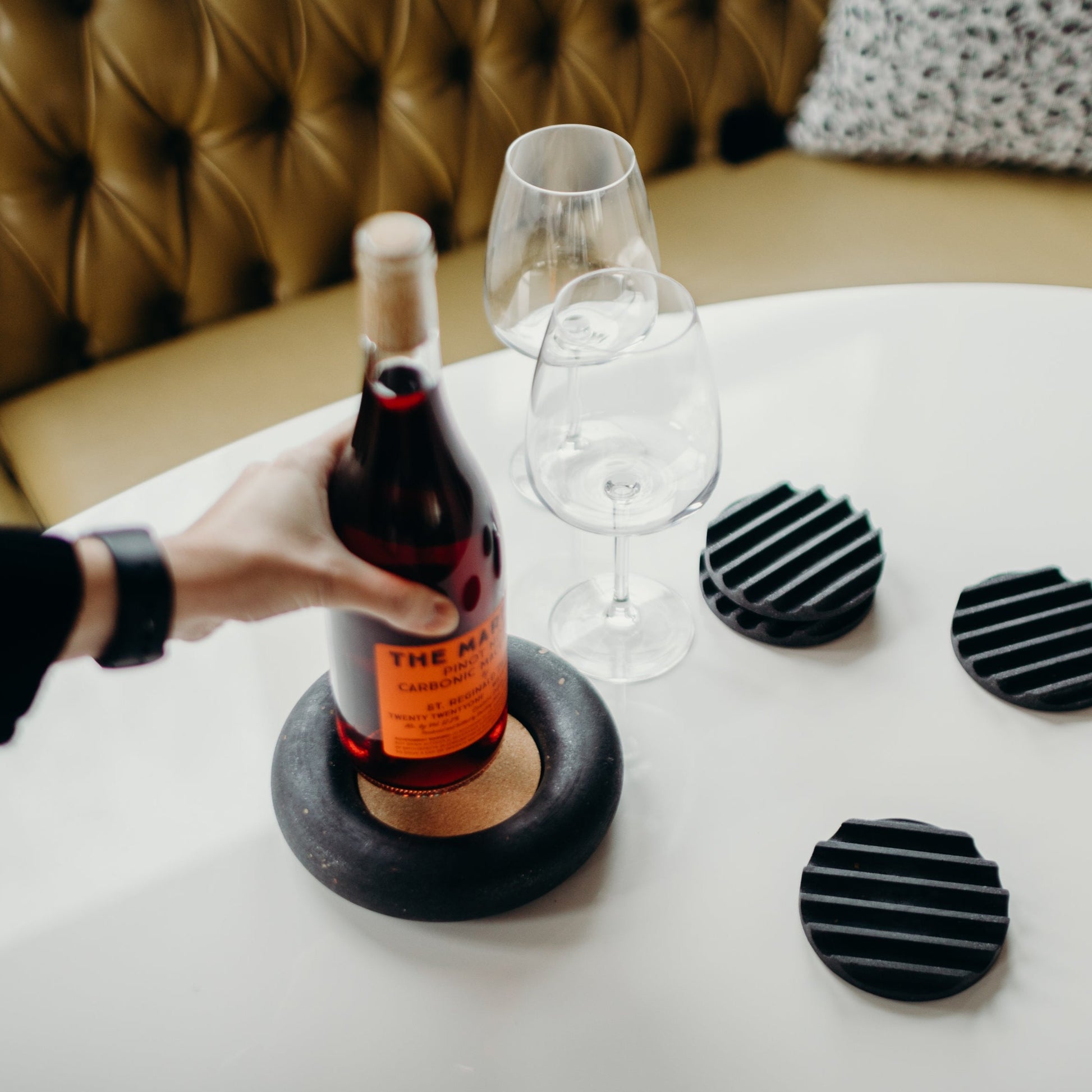This color photograph, captured in square format, showcases a detailed and realist representation of a wine-related setup. The central focus of the image is a wine bottle and two wine glasses arranged on a white-covered table with a rounded edge. The view is slightly from above, providing a clear look at the arrangement. 

A left hand, appearing to be of a young woman, reaches in from the left side of the frame. The hand, clad in a black sleeve, holds a wine bottle featuring a dark red wine and a cork at the top. The orange label on the bottle, though partly turned and not fully legible, displays text in black, including "Pinot" and partially "carbonic."

The bottle is being placed into a distinctive round coaster that mimics a tire with its black rubber raised edge. In the center of the table are two clear stemmed wine glasses positioned one behind the other. To the right of these glasses are four additional coasters with a black 3D zigzag or sawtooth texture, likely made from a rubber-like material.

In the upper part of the image, a beige booth with a diamond-tufted upholstered back and a throw pillow on the right is visible, adding context to the setting. The photographic lighting, sourced from outside the frame, highlights the texture and details of the objects, emphasizing the realistic style of the scene.